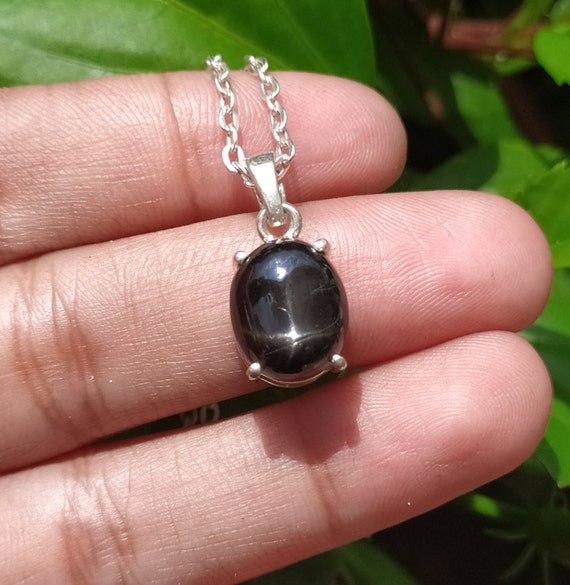In this close-up image, a person with light skin is holding up a necklace prominently featuring a pendant. The three middle fingers—the index, middle, and ring fingers—are delicately grasping the piece, with the index finger securing the chain and the middle finger supporting the oval-shaped pendant. The pendant itself is an elegant, polished gemstone with a dark gray hue, possibly an opal, encased in a silver clasp held together by four prongs. Sunlight glistens off the pendant and chain, casting a shadow on the person's hand and illuminating specks of dirt and dust. The background reveals a lush, green setting, filled with foliage and a noticeable brown stalk in the upper right corner. The vibrant outdoor light enhances the intricate details and reflections on the jewel, making it the focal point of the image.